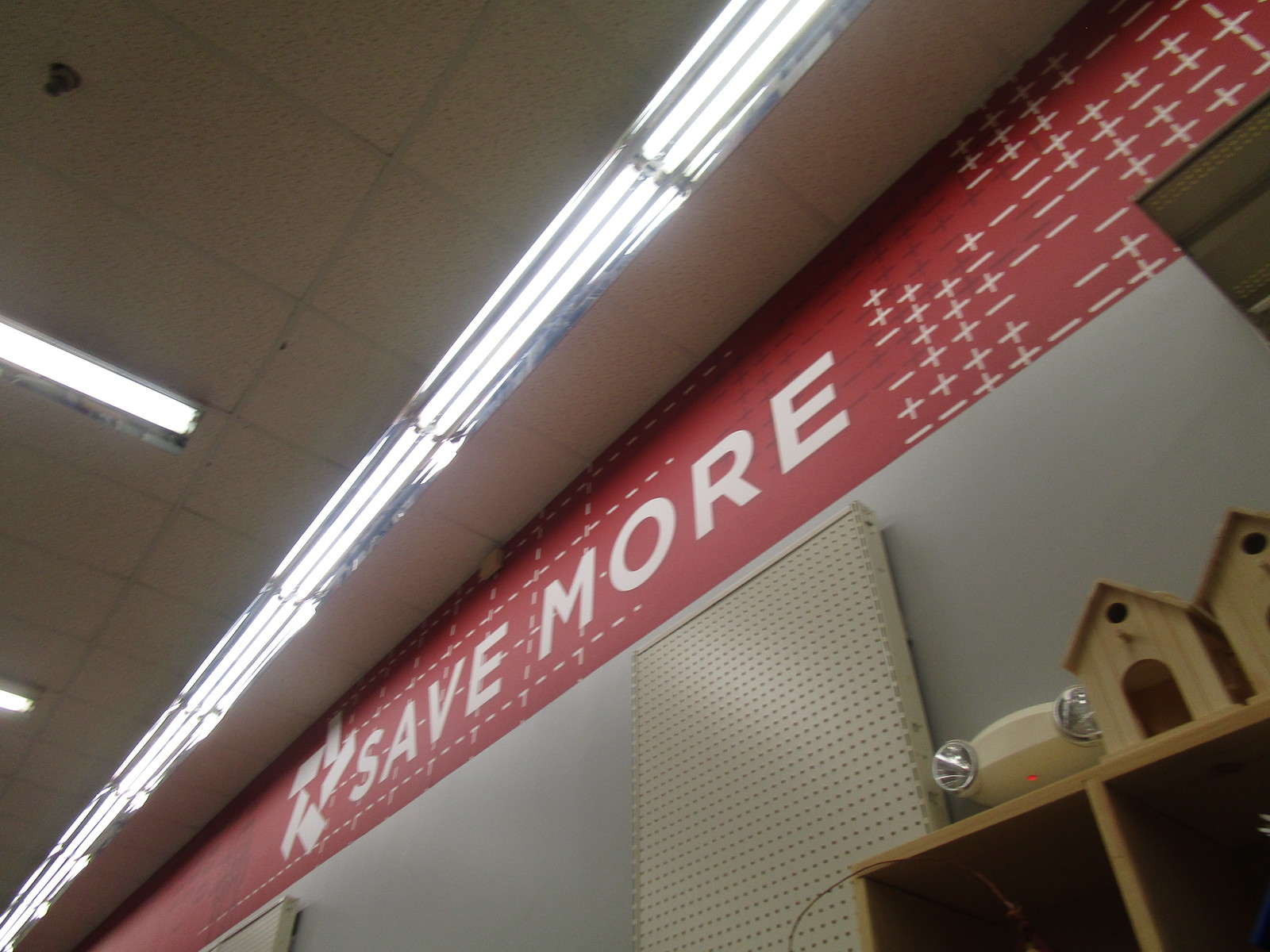In the photograph, taken from the interior of a store, the vantage point is distinctly upward, as if the viewer is looking towards the ceiling. The ceiling itself is commercial in appearance, comprising a grid layout of square tiles interspersed with rows of bright fluorescent lights. Dominating the space just below the lights is a prominent red sign with bold white lettering that reads, "Save More." Below this sign, an empty display rack is visible, designed for hanging items on hooks or peg hooks, though no merchandise is currently displayed. Towards the bottom right corner of the image, a wooden shelf is partially visible, holding several unfinished birdhouses, adding a touch of craft-like charm to the otherwise utilitarian scene.